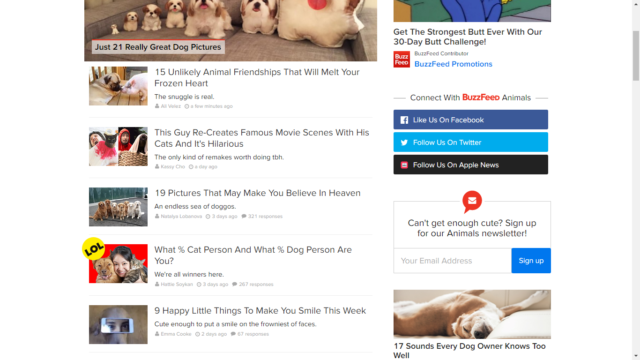The image captures a section of a webpage with a white background, featuring various elements and advertisements from BuzzFeed. Dominating the right side is a vertical, pale gray scrollbar, complete with the usual dark gray draggable section and directional arrows at both ends. The scrollbar is positioned near the top of its track.

In the top left corner of the webpage is a long, narrow photograph showcasing a row of ceramic figurine dogs. This image accompanies the title "21 Really Great Dog Pictures." To its right, there's a colorful rectangular graphic—composed of yellow, green, and blue geometric shapes—that promotes an article titled "Get the Strongest Butt Ever with Our 30-Day Butt Challenge."

Further down on the right side, there's a series of BuzzFeed promotional buttons for connecting with their animals section on social media: a dark blue "Like Us on Facebook" button, a light blue "Follow Us on Twitter" button, and a black "Follow Us on Apple News" button. Below these buttons, a thinly outlined rectangle invites visitors to sign up for the animals newsletter. Inside this rectangle, a red speech bubble housing an envelope icon encourages email subscriptions, with space to enter an email address and a blue sign-up button to the right.

At the bottom right, there is a photograph of a Shiba Inu dog lounging on its back, captioned "17 Sounds Every Dog Owner Knows Too Well."

On the left side, beneath the main photo of ceramic dog figurines, there is a vertical column of five thumbnails. Each thumbnail features an image related to dogs or dogs with people, accompanied by engaging, clickbait-style titles. The first thumbnail is titled "15 Unlikely Animal Friendships That Will Melt Your Frozen Heart," followed by similarly themed titles.